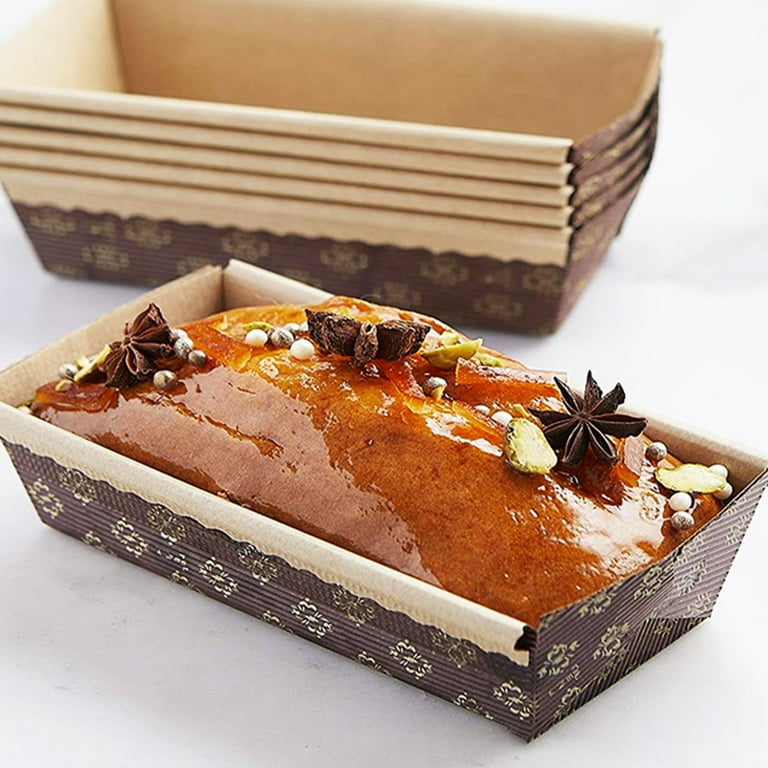The image showcases a delicious-looking loaf, which could either be a bread or a cake, sitting in a brown, boat-like, corrugated paper container. The loaf, with a rich brownish-red color that resembles a cinnamon bun before icing is applied, has a glossy glaze on top, indicating either a sugary syrup or sauce. Adorning the glaze are star anises, nuts, and chocolate-like decorations that add a touch of elegance. The photo's backdrop is a plain white surface, against which a stack of five similar, slightly out-of-focus paper containers is visible, indicating preparation for making multiple loaves. The overall impression is that the loaf might be featured in a retro-style cookbook, possibly from the 1960s or early 1970s, capturing a nostalgic culinary essence.